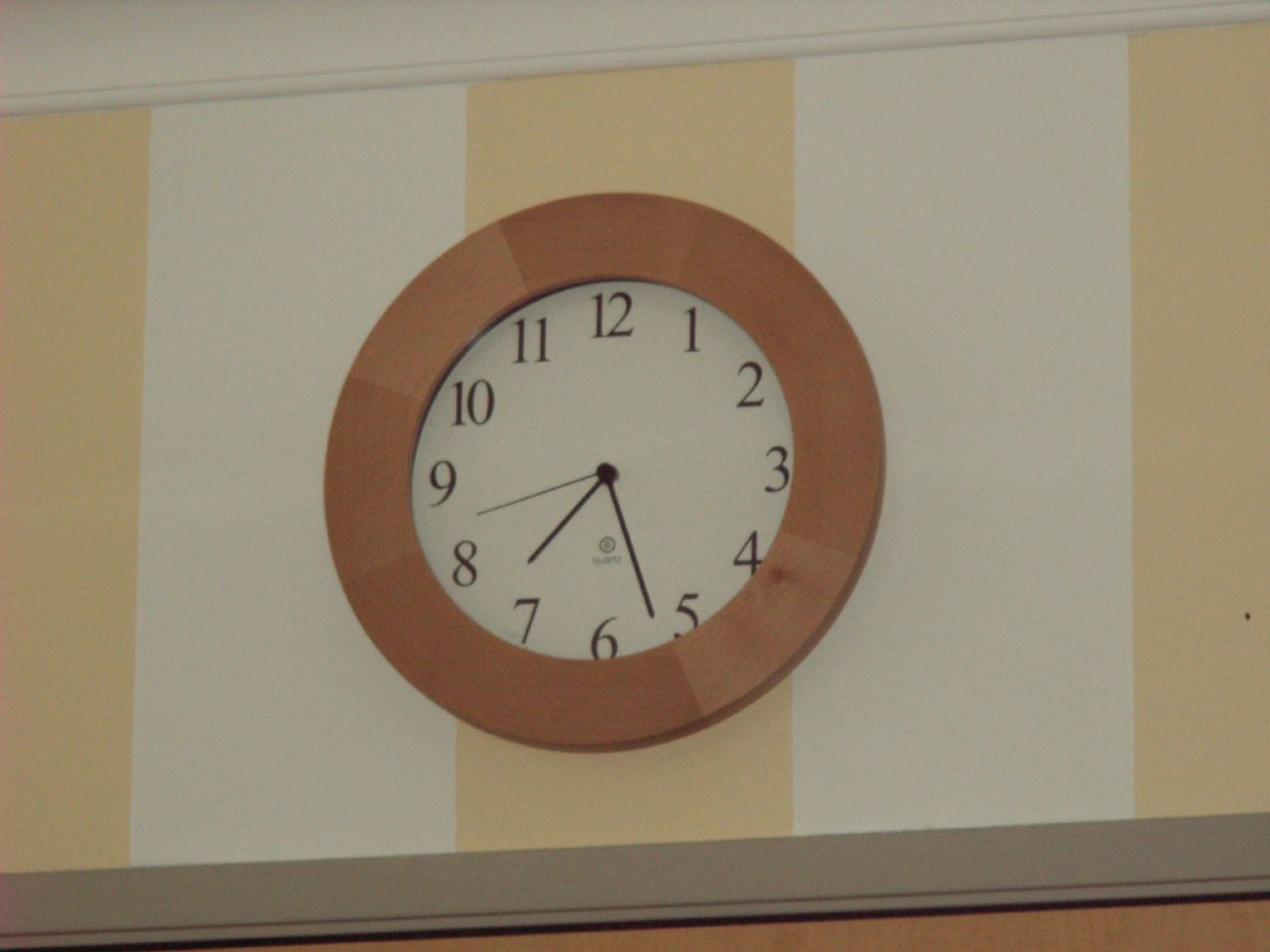The image depicts a clock with a brown wood rim, featuring variations that resemble maple. The clock face is white with black numbers from 1 to 12, and black hands for hours, minutes, and seconds. The time on the clock is approximately 7:32, with the minute hand between 5 and 6, the hour hand between 7 and 8, and the seconds hand between 8 and 9. The wall background consists of alternating vertical lines in white and light brown or tan, with additional dark brown and wood elements towards the bottom. The scene is slightly shadowed, suggesting it is not well-lit. The setting appears to be a commercial space such as a restaurant or a mall shop, though it could also be a home.